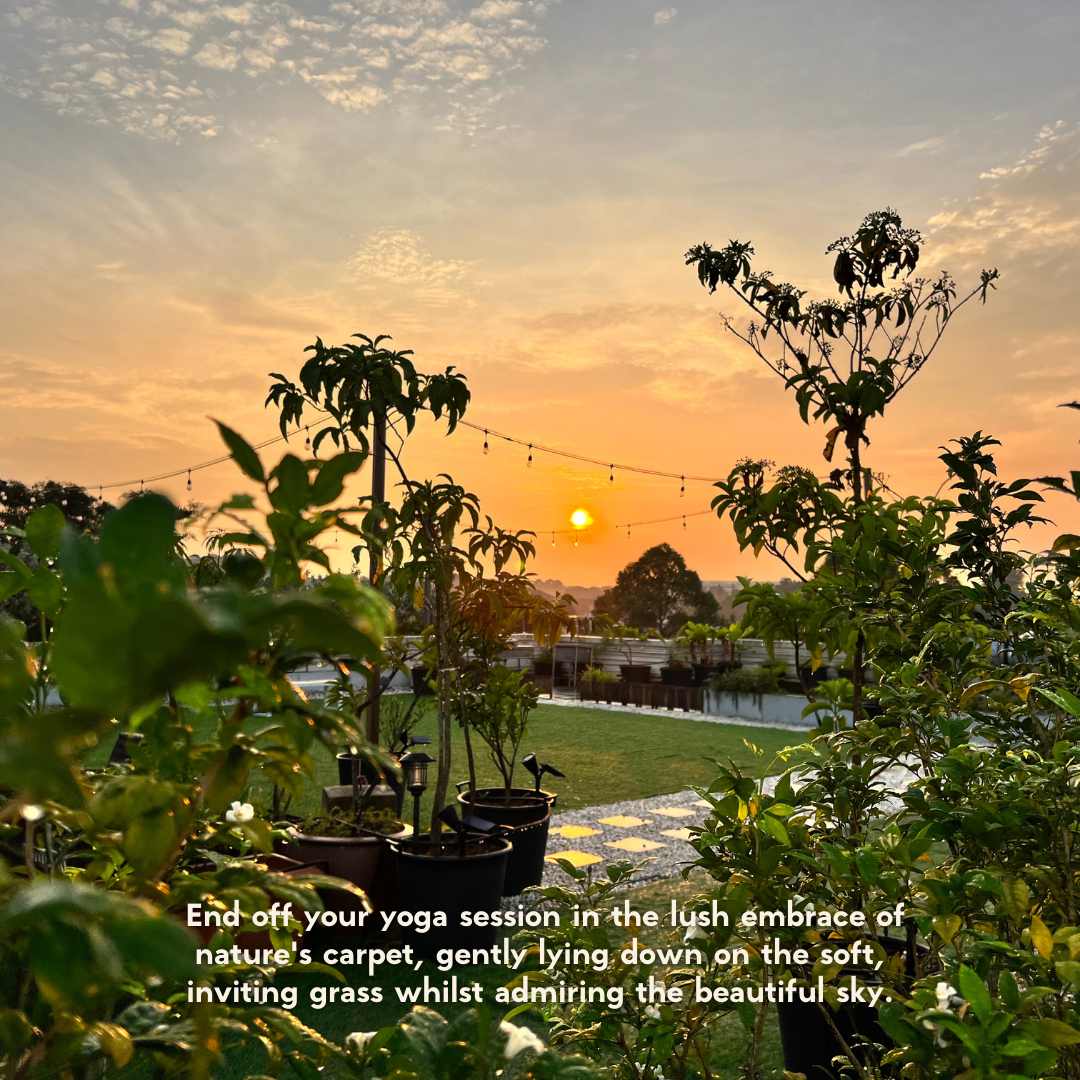The image captures a serene outdoor nature scene, potentially someone's backyard, during what appears to be a sunset. The sky transitions from a reddish-orange near the horizon to a clear blue higher up, with some faint clouds scattered throughout. The sun, positioned centrally, casts a warm glow over the landscape. In the foreground, there are potted plants, including one notable black pot, and a green grassy area bordered by a gray rock sidewalk and white rectangular stepping stones. Trees are abundant, framing a body of water in the distance—perhaps a river or pond—with buildings visible further back. Suspended overhead is a string of festoon lighting or possibly an electric cable, attached to a pole. The entire scene is bathed in the soft, inviting hues typical of dusk, completed with the caption at the bottom: "End off your yoga session in the lush embrace of nature's carpet, gently lying down on the soft inviting grass whilst admiring the beautiful sky."